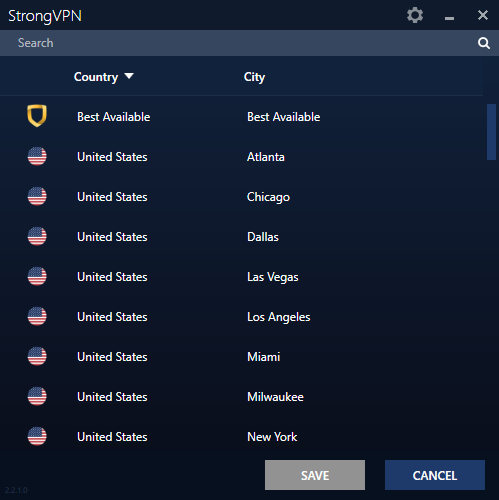The image depicts a user interface for a VPN (Virtual Private Network) application. Dominating the interface is a black square with the phrase "Strong VPN" written in white text. Above this text, there's a gear icon, an underline, and a close button represented by an 'X'.

Below this header, there is a search bar in a light gray shade with the placeholder text "Search" in an even lighter gray. To the right end of the search bar is a white magnifying glass icon.

The UI is divided into two columns - one labeled "Country" with a drop-down triangle and the other labeled "City". Beneath the column headers, there's a gold shield icon, and under both "Country" and "City", it says "Best Available".

Following this, eight rows display the flag of the United States, with "United States" written next to each flag. Next to each instance of "United States", the corresponding cities are listed: Atlanta, Chicago, Dallas, Las Vegas, Los Angeles, Miami, Milwaukee, and New York.

At the bottom of the interface, there are two buttons: a gray "Save" button with white text, and a blue "Cancel" button also with white text.

This interface allows the user to select the best available VPN server based on their location, presumably to optimize their internet browsing experience with the VPN.